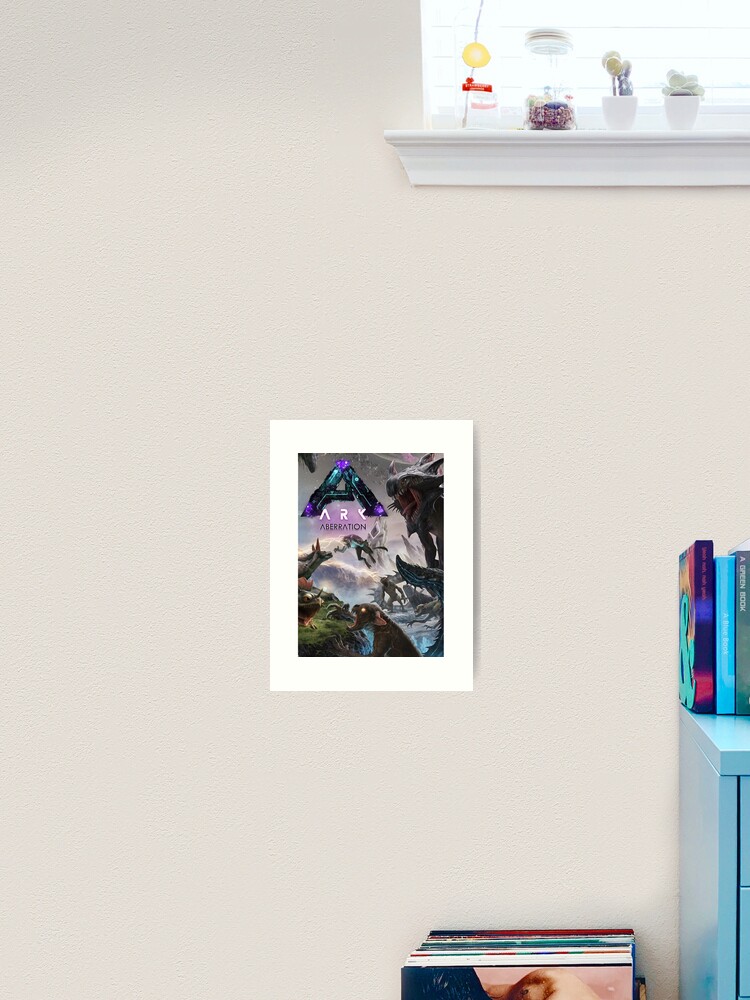This photo captures a section of a tan-colored interior wall in a home. Dominating the center of the image is a small poster, possibly 8 by 10 inches in size, bordered in white. The poster features graphic art with the word "ARK Aberration" written in white letters, accompanied by a prominent fluorescent blue and purple 'A'. The artwork displays various fantasy animals, including dinosaurs, dragons, a little flying creature, and a wolf-lion hybrid, suggesting it might be computer-generated or inspired by video game art.

Above the poster, at the very top of the image, is a bright, sunlit window with a white sill, adorned with a couple of succulents and a jar, possibly containing another plant. Blinds partially cover the window. To the right of the poster, the edge of a light blue chest of drawers is visible, topped with books held in by teal bookends. Below the drawer, one can discern the top edges of magazines or record albums placed on their side in a holder. The rest of the wall is bare, highlighting the poster as the focal point of this cozy, sunlit space.